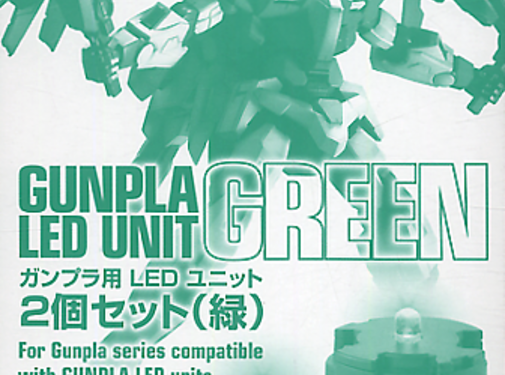The image is an advertisement for a Gunpla Green LED Unit, predominantly featuring green and white colors. Central to the image are the words "Gunpla Green LED Unit," with parts of the text showing a white outline. The background is white, providing a clear contrast to the vivid green text and objects.

Towards the right edge of the image is an incomplete text reading "for Gunpla series compatible," indicating the LED unit's compatibility. There is prominent use of Japanese or Chinese characters, alongside English words such as "LED" and the numeral "2," implying a set of two LED units.

The background also partially features a green figure, which appears to be a robotic character or Gundam figurine standing with legs spread apart and holding items in both hands. The upper extremities and head of this figure are cut off from the frame, creating a dynamic, athletic pose. In the bottom right-hand corner, there is a green platform with an illuminated LED light bulb. This LED unit and platform further emphasize the product being advertised.

Overall, the image blends textual details in green impact, bubble fonts, and illustrations of the LED unit and a robotic figure, creating a vivid, high-contrast advertisement.